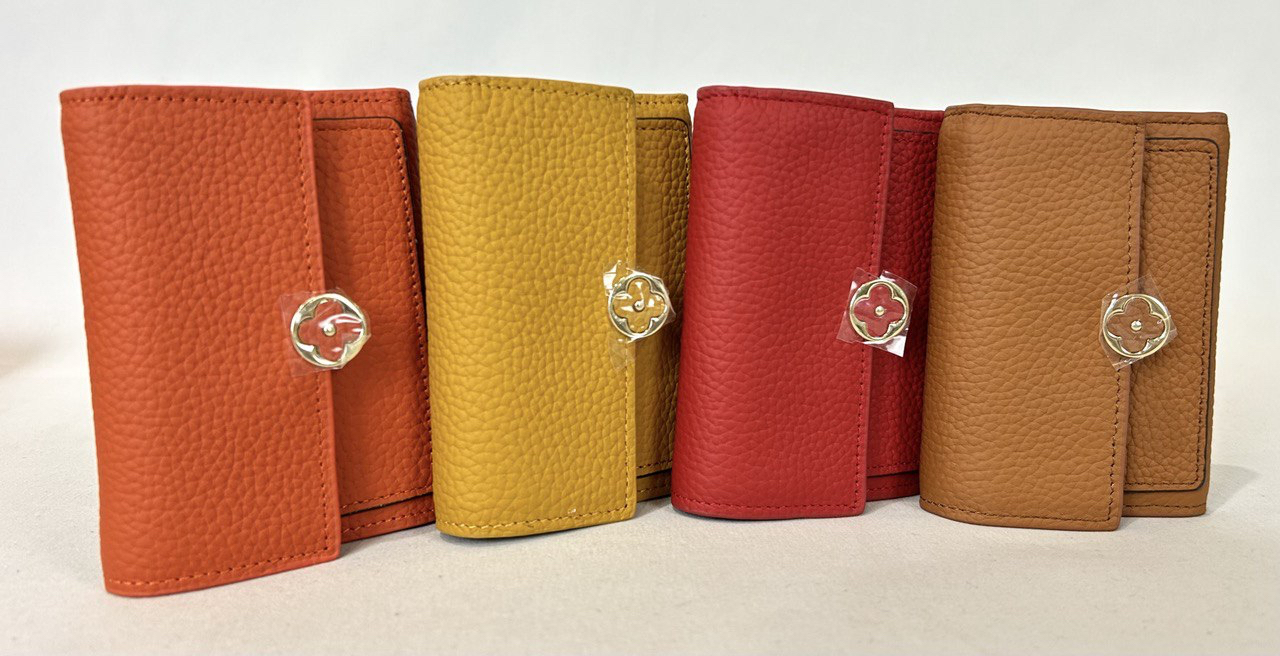The image is a well-lit product photograph showcasing a collection of four rectangular women's pocket books, also described as small clutches or wallets, arranged standing on their edges in a row against a pristine white background and foreground. These pocket books, which appear brand new and made of leather, feature a simple yet elegant design with a flap closure. The flap is secured by a distinctive silver clasp that resembles a four-petaled flower or clover, adorned with a rose pattern. This silver clasp on each pocket book is covered in protective plastic. The colors of these pocket books are, from left to right: orange, mustard yellow, red, and brown. The pocket books are displayed in a diagonal arrangement, partially overlapping each other, with the brown one fully visible at the end. Despite the high-quality lighting, the photograph might be slightly out of focus. There is no text or other distractions in the image, directing full attention to the pocket books' design and colors.